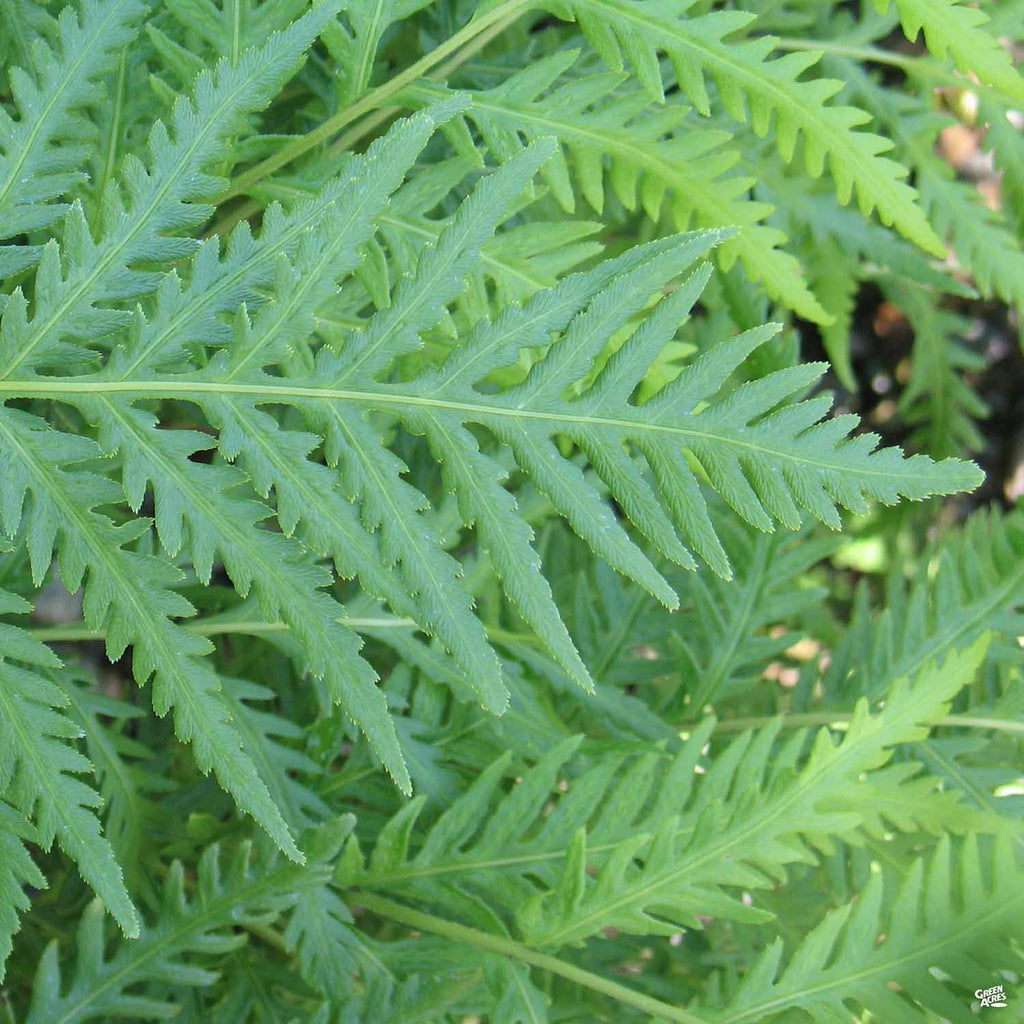This is a close-up, color photograph taken outside during the day, which fills the entire frame with the segmented, needle-like fronds of a pale green fern-type plant. The fronds extend from left to right, top to middle, and bottom left up to the center, creating a detailed and intricate pattern. The top and bottom of the image allow light to shine through, adding depth to the photo. A slight blurring is visible in the far-right top background, keeping the focus on the plant's intricate fronds. The text "green acres" is subtly positioned in the bottom right corner. The image captures just the plant leaves, with no flowers or other elements present, offering a pure and serene view of nature.